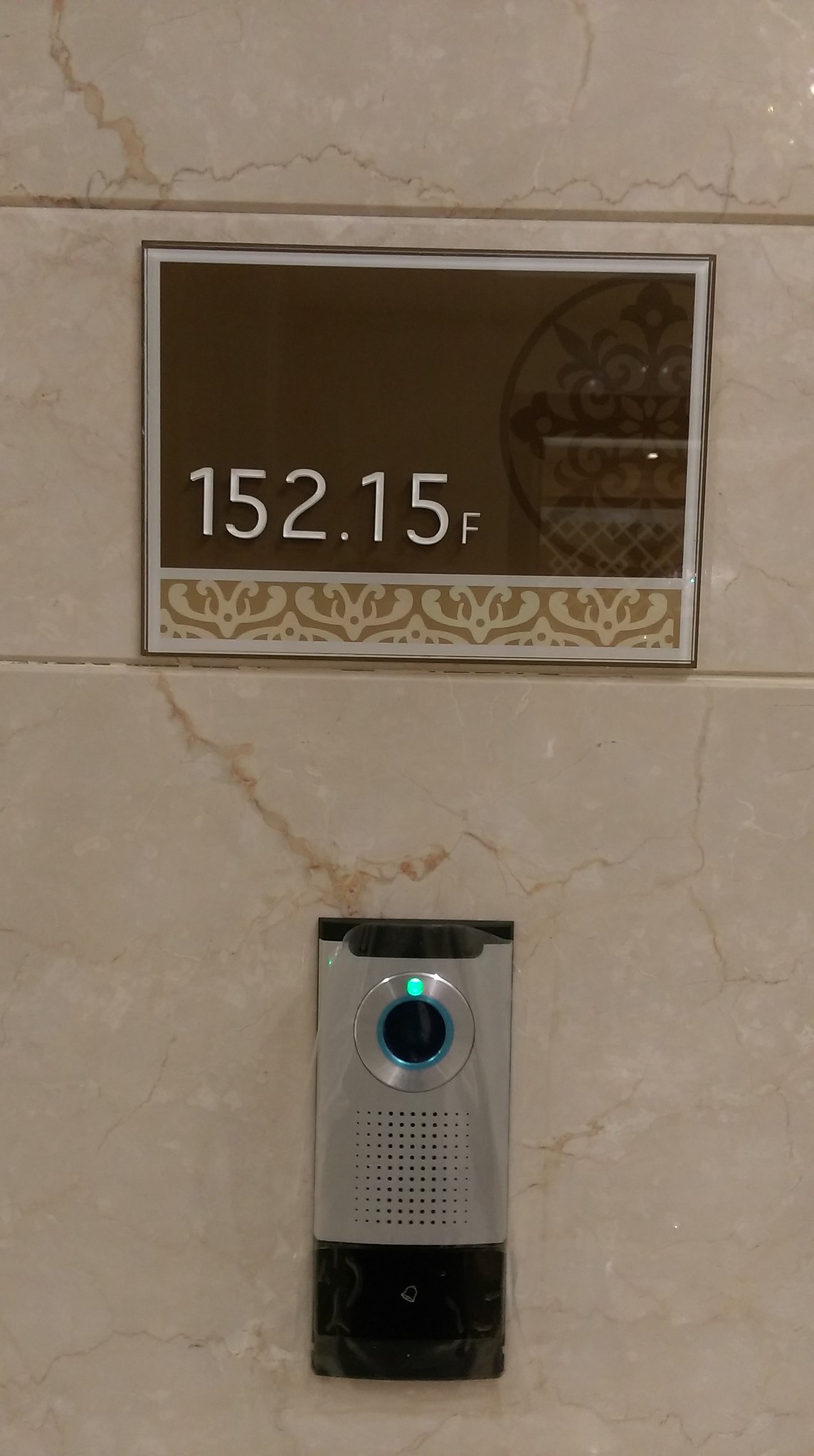Photograph showcasing a close-up view of a section of a marble wall with distinct cream and brown streaks. In the foreground, a stylish dress drapes partially over a dark brown plaque, which has intricate white-trimmed edges accompanied by decorative scrolling at the bottom. The plaque prominently displays "152.15F" in bold white lettering. Positioned vertically below the plaque is a sophisticated doorbell featuring a sleek black base and a silver body. A noticeable silver circle encloses a black area near the top, lit up by a small green dot. Above the circle sits a slender black trim, while below it, tiny perforations hint at the speaker’s presence, adding a practical yet elegant touch to the scene.